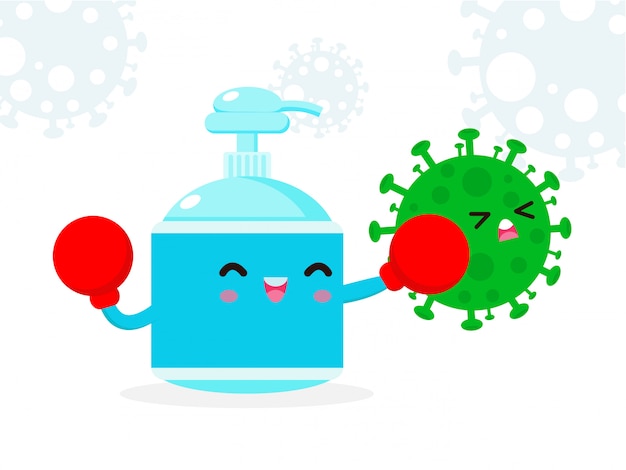This image is a charming and playful health-themed cartoon in a kawaii cute emoji style, likely inspired by Japanese or Korean illustration aesthetics. At the center of the image is an anthropomorphic hand sanitizer pump bottle colored in Tiffany blue with a lighter blue plunger. The bottle features a smiling face, complete with black closed eyes, pink cheeks, and a pink mouth displaying upper teeth. It extends cartoonish blue arms, each donning a round red boxing glove. 

The scene depicts the hand sanitizer in action, punching a large green virus. The virus, with its eyes squinted and a distressed mouth revealing white teeth, appears to be reeling from the impact of the punch. The virus is illustrated with signature spike proteins.

In the background, on a predominantly white canvas, there are faint gray watermark-like imagery of additional viruses, reinforcing the public health message. These subtle virus outlines suggest that they are being subdued or disinfected. The overall composition and clean, minimal color palette enhance the straightforward and engaging message to use hand sanitizer to fight against viruses, presumably during the COVID-19 outbreak.